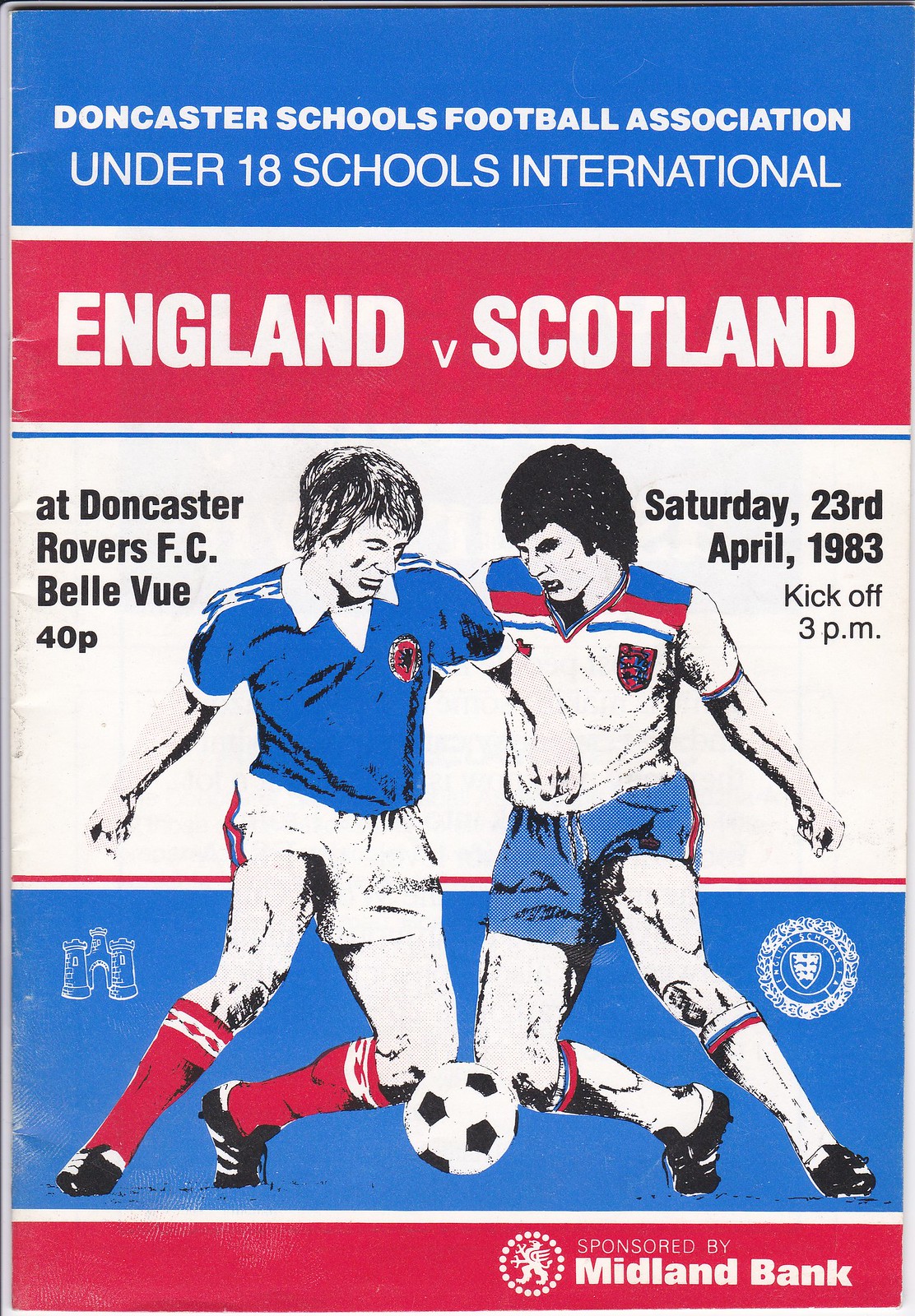This rectangular image is the front cover of an old-fashioned soccer program for the Doncaster Schools Football Association Under 18 Schools International match. The cover is designed in red, white, and blue colors. At the top, there is a blue bar with white text that reads "Doncaster Schools Football Association Under 18 Schools International." Below that, a red band with white text announces "England versus Scotland." Further down, a white band with black text provides details: "At Doncaster Rovers FC Bellevue, 40p Saturday 23rd April 1983 kickoff 3 p.m." 

The central part of the cover features an illustration of two young soccer players. The player on the left wears a solid blue shirt, white shorts, and red socks, while the player on the right dons a white shirt with blue and red highlights, blue shorts, and white socks. They are depicted mid-action, both vying for a black and white soccer ball positioned between them. Near the bottom, another red band with white text indicates sponsorship by Midland Bank, complete with its logo. The program cover also includes small additional graphics such as a pair of binoculars and a possibly indistinct logo related to Doncaster Schools.